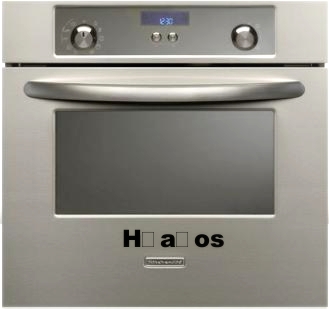The detailed image depicts a stainless steel oven with a distinct design. At the top, there's a horizontal rectangle housing a dark steel-colored inset rectangle. Within this inset, there's a small, horizontal window with a blue LED display showing the time 12:30. Below the display are two unnamed buttons. Flanking this central section are two large silver knobs; the left knob is marked with a timer ranging from 0 to 60, while the right knob likely controls the temperature.

The oven door, positioned beneath this control panel, features a semicircular stainless steel handle that spans the width of the door, allowing it to be opened easily. This door has a horizontal rectangular window, which appears dark and possibly opaque, or simply not in use. Below this window are black markings: the capital letter "H", a sketched rectangle, the lowercase letter "a", followed by another sketched rectangle, and finally the letters "OS". An unreadable name tag is located beneath these letters.